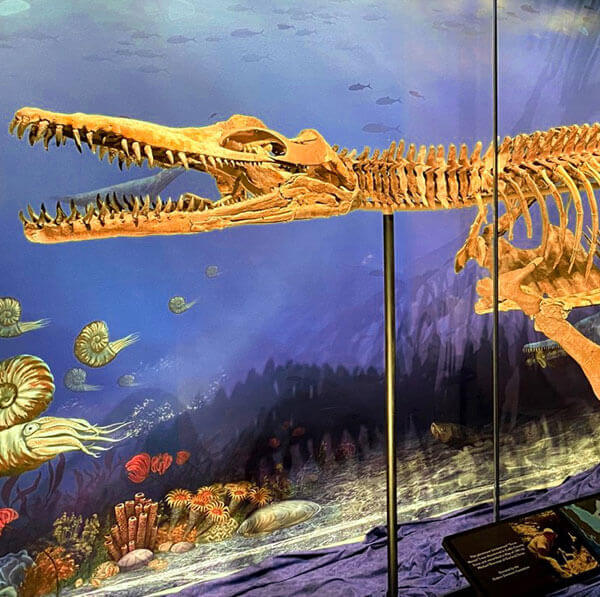This highly detailed image showcases a photograph or a photorealistic image of a fossil display, likely housed in a Natural History Museum. The fossil appears to represent an ancient undersea creature, potentially a prehistoric aquatic reptile or a dinosaur, resembling an alligator or crocodile due to its elongated jaw filled with sharp, prominent teeth. The head is oriented towards the left side of the image near the top half, featuring large eye sockets, while the body stretches towards and off the right side, revealing a visible spine with protruding ribs and part of a fin.

The fossil is supported by a tall black pole, which is anchored into blue fabric flooring, giving the impression of an underwater scene. The backdrop enhances this aquatic illusion, painted with hues of blue and depicting corals and anatomies in gold and yellow. There are also white squids and other marine creatures drifting off to the left, adding depth and context to the display. Positioned at the bottom left of the image is a black plaque with textual information and illustrations, though the details are obscured and unreadable due to the image resolution. The overall scene is contained within a glass display, emphasizing the fossil’s importance and likely educational purpose in illustrating the evolution of ancient sea creatures and dinosaurs.